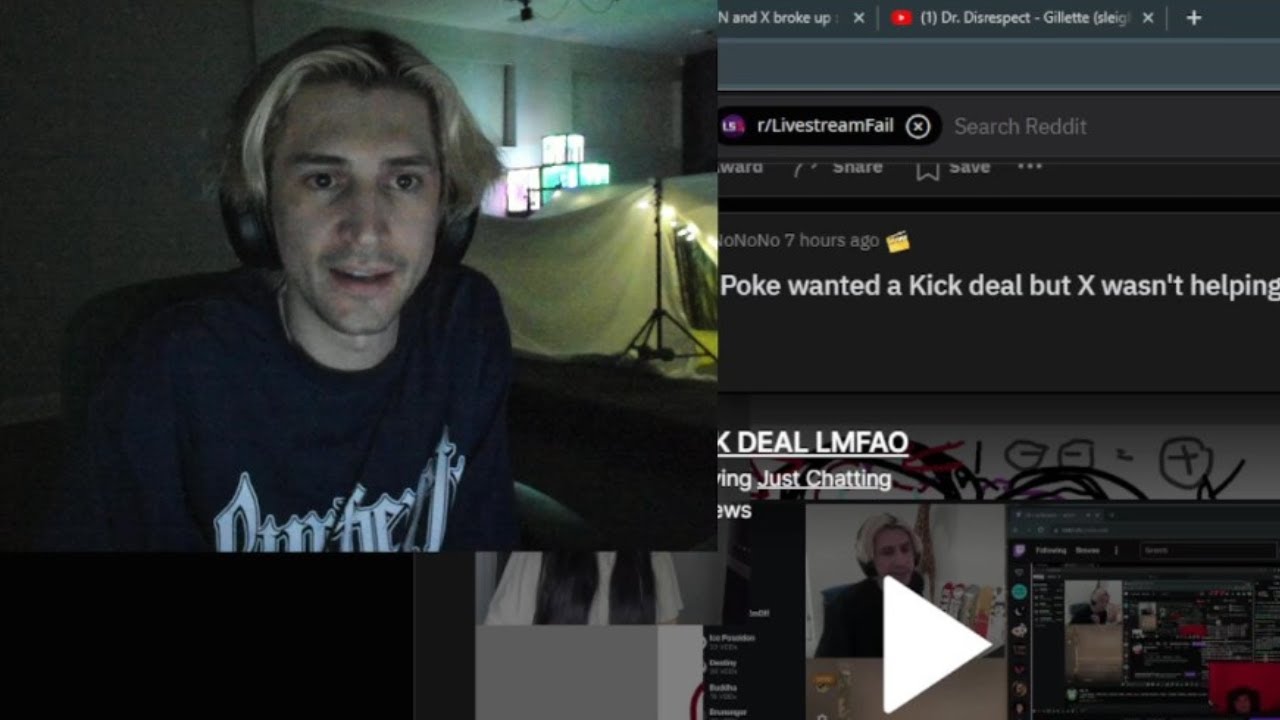A computer screen displays an image of a man in the upper left corner, likely during a live stream. The man is wearing a black t-shirt with white print near the top and has blondish-brown hair along with some facial hair. Behind him, lights are set up and there is a beige divider visible. Along the right side of the screen, various text elements are shown, including "live stream fail" or "r/LiveStreamFail," followed by a search bar labeled "Search Reddit." Further down, it reads "No No No - 7 hours ago," referencing a user named "Poke" who wanted a kick deal that "X wasn't helping." There are arrows pointing in different directions alongside additional text such as "Deal LMFAO" and "Just Chatting."